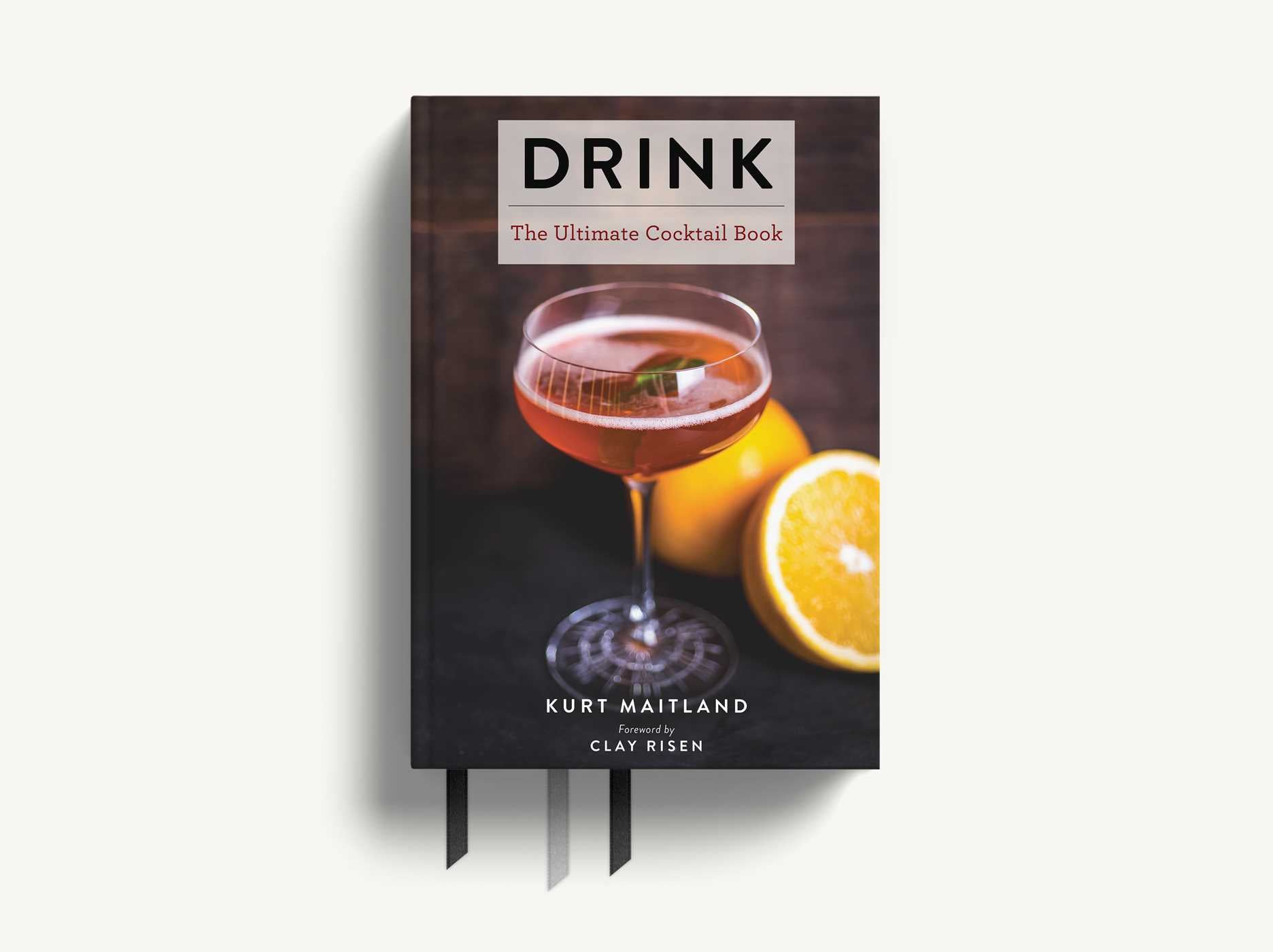The image features the cover of a book titled "Drink: The Ultimate Cocktail Book" by Kurt Maitland, with a foreword by Clay Risen. The cover showcases a champagne coupe glass filled with a reddish-pink beverage, accented by a ring of foam around the liquid. Floating within the drink is a small, square-shaped object, which could be a piece of candy or fruit. The glass is set against a dark background, with two blurred orange slices in the backdrop—one slice facing the viewer showing its rind, and the other displaying the juicy flesh. The detailed and contrasting colors of the red drink and the orange slices stand out against the otherwise simple, dark backdrop. Additionally, the book is shown resting on a gray surface, with three bookmarks—two black and one gray—hanging from the bottom.